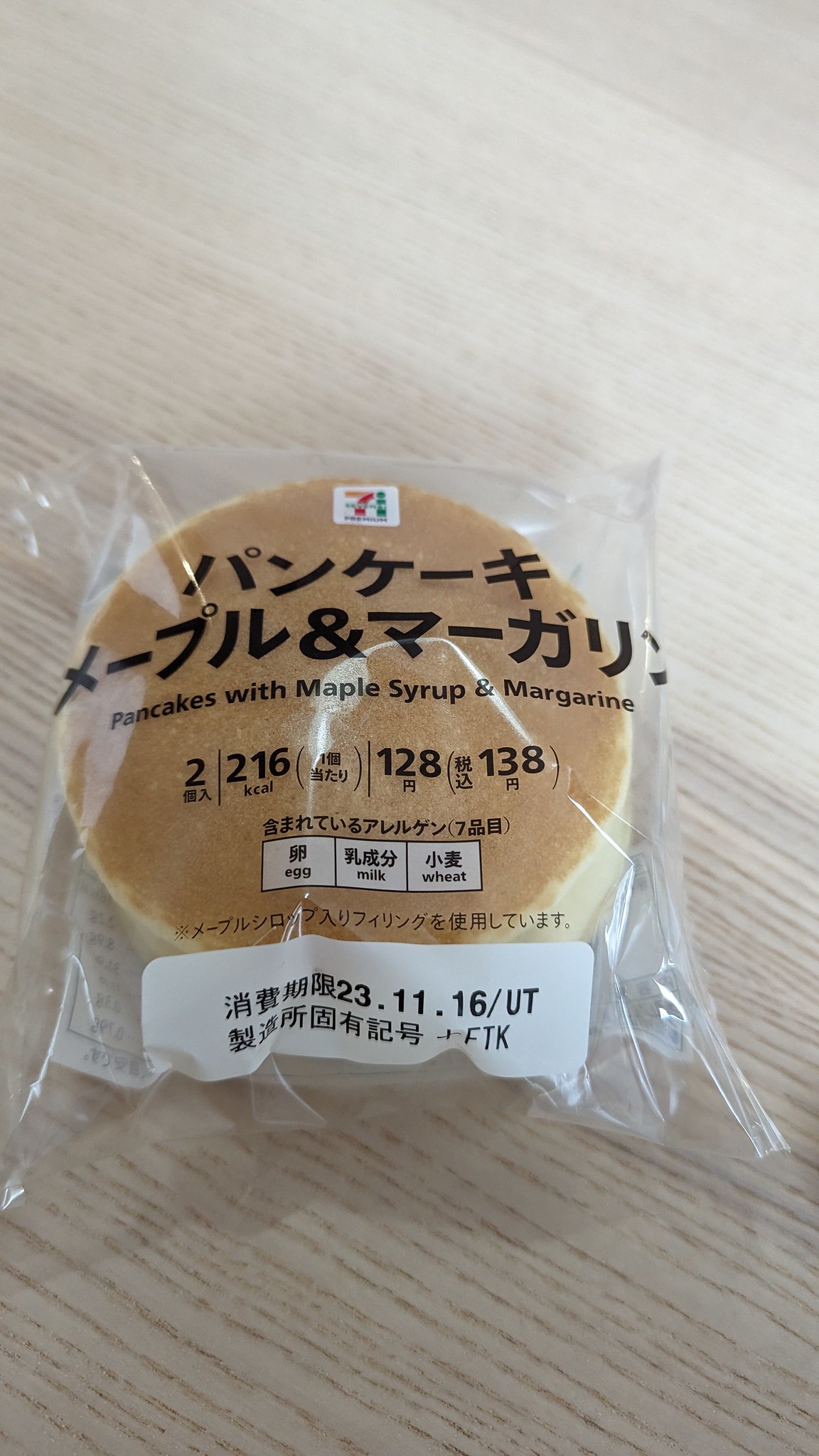The image depicts a package of pre-made pancakes, most likely from a 7-Eleven in an Asian country, discernible from the Japanese writing on the clear plastic wrapping. The package contains a stack of several small pancakes, which have a brown top and white sides. Prominently written beneath the Japanese characters are the English words: "Pancakes with Maple Syrup and Margarine," indicating that the pancakes are already infused with these ingredients. Detailed nutritional information such as calorie count, fat, sodium levels, and other ingredients are listed below in a mix of English and Japanese text. The pancakes are wrapped in plastic designed for microwaving, with the entire package sitting on a fake wood countertop. The multilingual packaging shows the convergence of Japanese and Western cuisine elements, alongside the recognizable 7-Eleven logo situated at the top of the package.